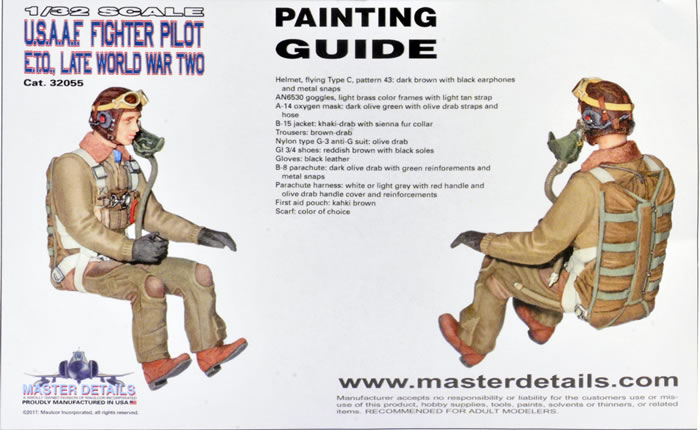This image features a detailed painting guide for a 1:32 scale figurine of a late World War II USAAF fighter pilot in the European Theater of Operations (ETO). At the top center, bold black letters prominently display the title "Painting Guide." In the upper left corner, white text specifies, "1:32 scale, USAAF fighter pilot, ETO, late World War II," accompanied by images of the pilot figure. The figure appears seated, as if in an airplane, though no chair is visible. The pilot wears a greyish-tan flight suit with brown shoes, a brown aviation cap with goggles positioned on the forehead, and a green oxygen mask hanging loosely from his face. His hands are encased in black gloves. 

On the right side of the guide, an image shows the back of the figurine, including brown hair or helmet, a backpack, and the same brown shoes. Additional details such as "helmet flying type C pattern 43, dark brown with black earphones and metal snaps" further elaborate on the figurine's attire.

The guide also includes logos and text on the left side, such as a plane logo and the brand "Master Details," along with the phrase "proudly manufactured in USA." The bottom right corner features a website, "www.masterdetails.com," and a disclaimer absolving the manufacturer of responsibility for the customer's use or misuse of the product.